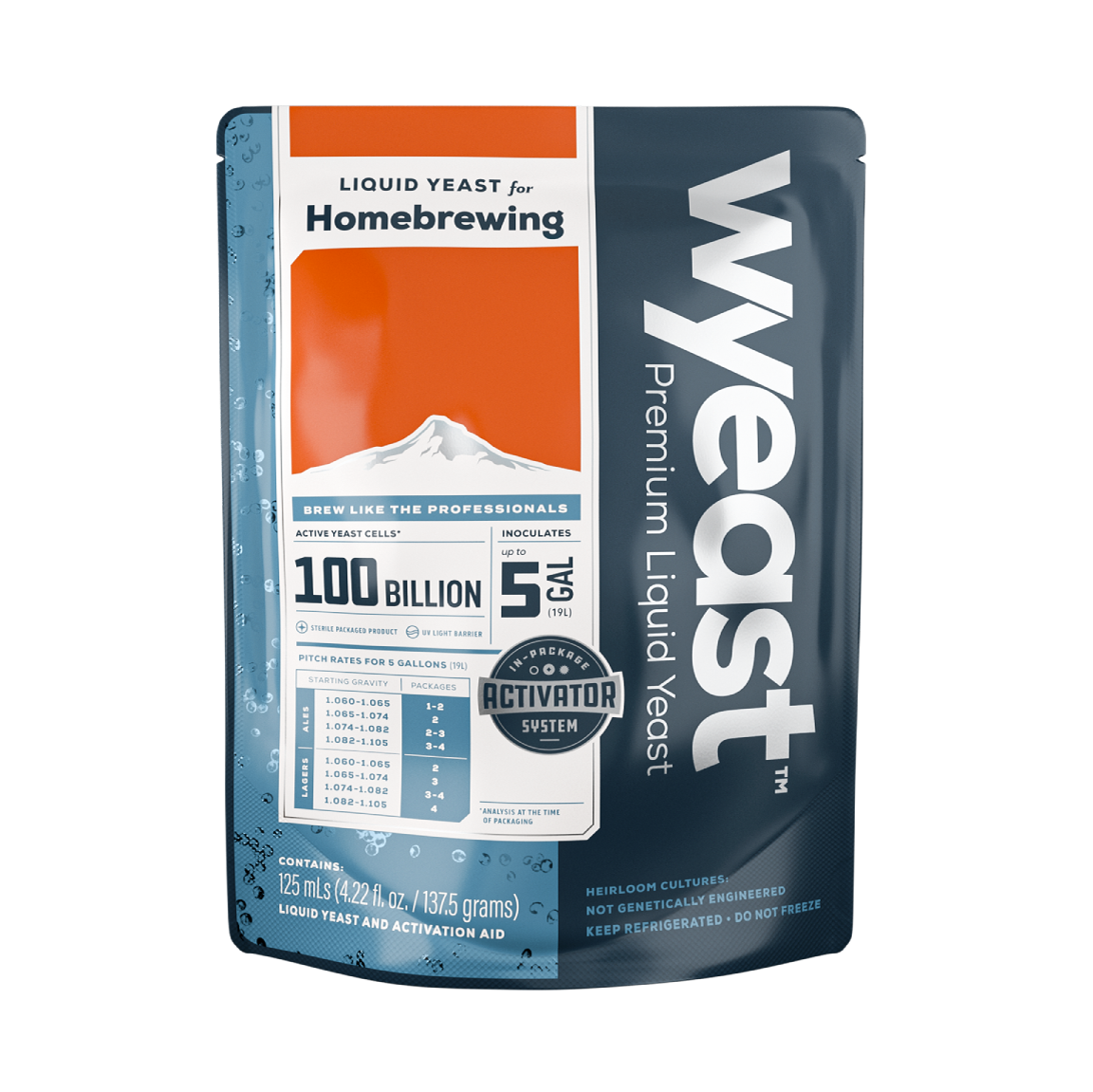This is a modern-looking cellophane package of yeast, primarily designed for home brewing. The package features a striking two-sided design with dark blue on the right and a white label with an orange top on the left. On the right side, large white text reads "W-Y-E-A-S-T" vertically, accompanied by smaller white text underneath that reads "Premium Liquid Yeast." 

The left side showcases an illustration of a snow-capped mountain against an orange sky. A white bar with black text stretches across the top, reading "Liquid Yeast for Home Brewing." Beneath this, in smaller blue print, it says "Brew Like the Professionals." Additional text on this side indicates that the yeast contains 100 billion active yeast cells capable of inoculating up to five gallons. Details also include specific measurements of the content: 125 milliliters (4.22 fluid ounces or 137.5 grams).

The package highlights several features: "In-Package Activator System," "Sterile Packaged Product," and "UV Light Barrier." There's also a chart and text providing pitch rates for five gallons. At the very bottom, it reiterates that this is a "Liquid Yeast and Activation Aid." The background on the left side also features a light blue area with metallic-looking bubbles, adding to the package's modern aesthetic.